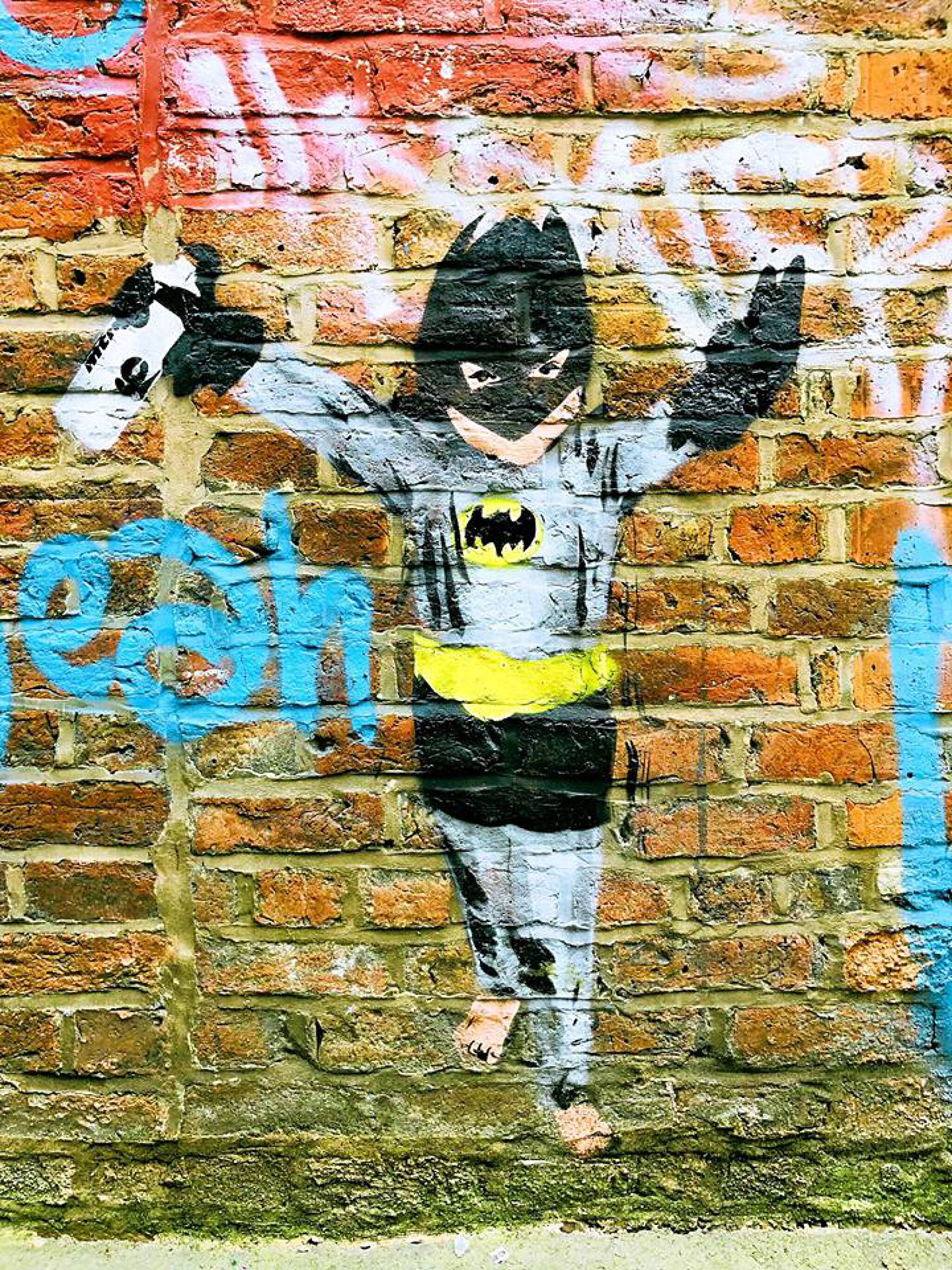A detailed piece of graffiti art adorns a red brick wall, prominently featuring a young boy dressed in a Batman costume. The boy wears the iconic black Batman mask with its two pointed ears and eye holes, a black shirt with the Batman emblem in the center, and a traditional yellow utility belt. He is also dressed in gray pants, black shorts, and black gloves, but notably, he is barefoot. His arms are outstretched, holding a white can with the number '94' on it, suggesting he might be the graffiti artist responsible for the work. Surrounding him, the wall displays various other graffiti elements, including smears of red paint at the top and white and blue spray-painted letters. The lower part of the wall appears weathered and mossy, adding to the gritty urban aesthetic. Despite the detail in the artwork, there is no visible signature of the artist.